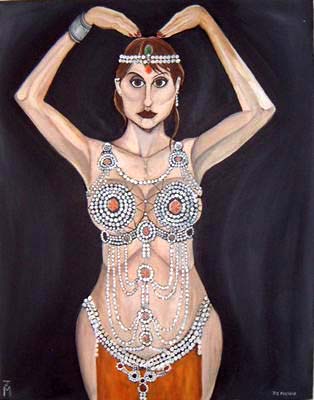The painting portrays a woman with light skin and brown hair, adorned with a white pearl headband around her forehead and a red bindi. She has her arms raised, fingers delicately touching her hair, adopting a pose reminiscent of a dancer or a genie. Her sharp facial features include a long nose and maroon-colored lips. She is dressed in a revealing outfit comprised mainly of pearls and jewels, with a see-through bra that barely covers her large breasts, featuring circular arrangements of pearls and central red jewels. Dangling jewels descend from her breasts over her stomach, and her lower body is modestly covered by an orange cloth adorned with jewels of black and red hues. She also wears a grey bangle on her right wrist. Decorative pearl strands extend across her outfit, which shows off her figure in an explicit manner. The background of the painting is entirely black, providing a stark contrast to her jewel-embellished attire. Notably, a small signature of the painter is visible in the lower right corner, and a logo is present at the lower left.